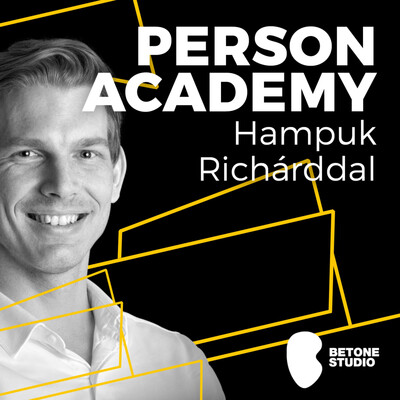The black and white photograph features a fair-haired, white man smiling subtly at the camera, with his head and left shoulder slightly angled away. He is wearing a light-colored button-down shirt and has a very short mustache. The image is set against a pure black background, with geometric yellow shapes, including parallelograms and lines, superimposed both behind and in front of him. The man occupies about the left half of the image, while to the right, white blocky text in all caps reads "PERSON ACADEMY." Below this, smaller text identifies him as "Hampuch Richardal." In the bottom right corner, a white, blob-like logo with the text "B-Tone Studio" in small block letters completes the design.